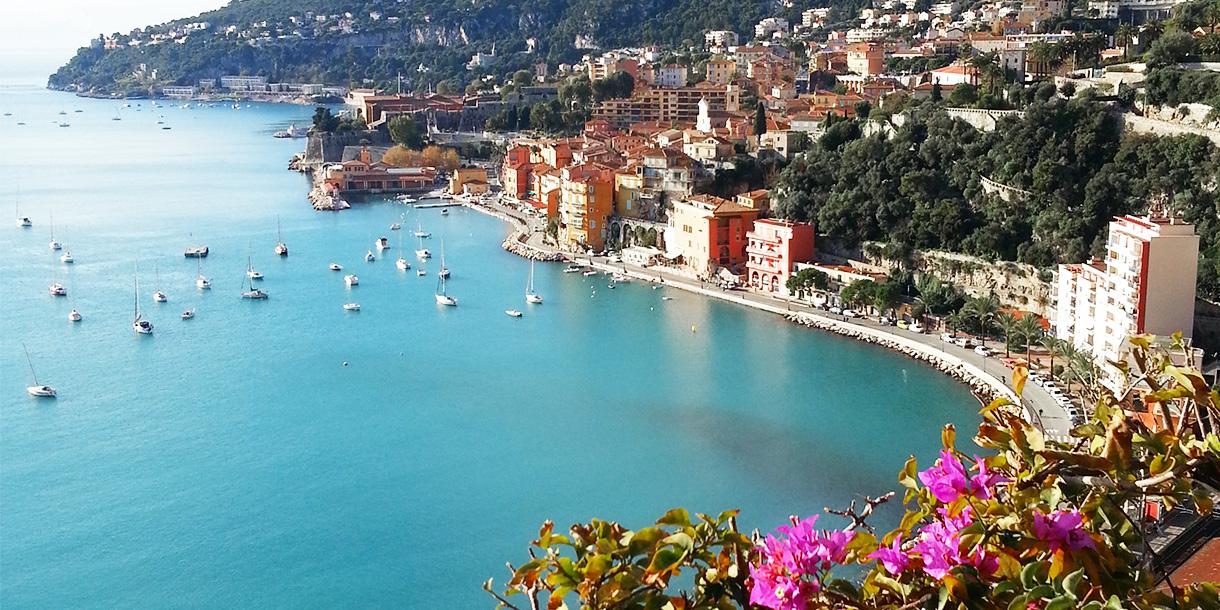This aerial landscape photograph captures the vibrant coastline of a bustling town situated within a picturesque bay. The central focus is the deep aquamarine waters of the bay, speckled with an impressive array of at least 20 sailboats, appearing stationary as if leisurely anchored. The left side of the image is dominated by this blue expanse, while the bottom right foreground features lush greenery adorned with eye-catching purple fuchsia flowers.

A street runs parallel to the shoreline, where you can spot a few parked cars and pedestrians, emphasizing the area’s civilized, tourist-friendly nature. Along the immediate coast, a combination of towering structures, possibly hotels, apartments, and assorted establishments, rise up to 12 stories high, flanked by verdant trees and palm trees, signaling a warm and thriving climate.

Extending back from the beach, the landscape transforms into hilly terrain densely packed with more residential buildings and rich greenery. The upper portions of the photo, particularly the top center and upper right, showcase this mountainside development, dotted with the white specks of distant buildings amidst the foliage. The photo, clearly taken from a significant altitude—likely from a mountaintop—provides a grand, sweeping view of this vividly diverse and well-constructed coastal area.